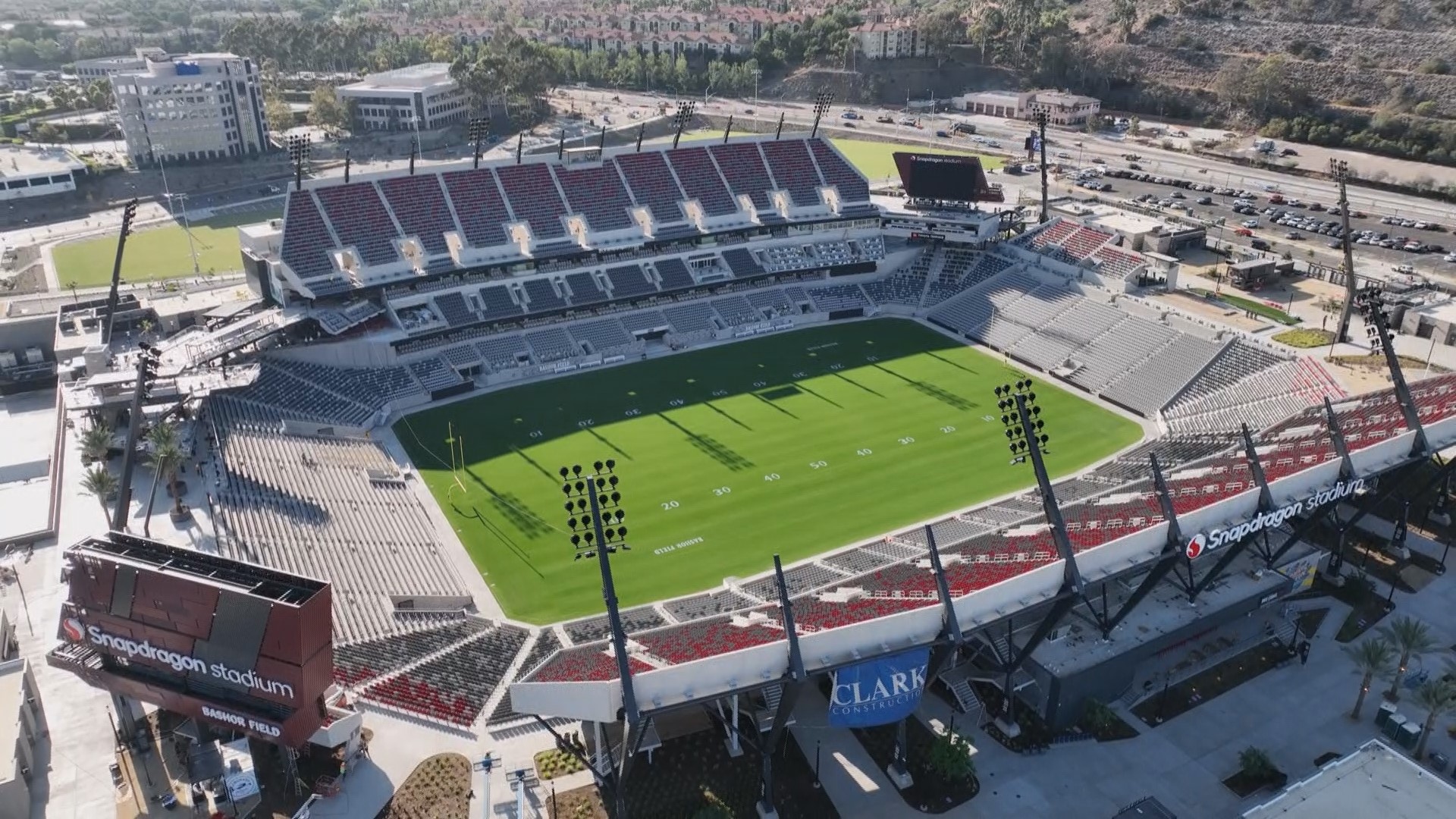The image is an aerial view of Snapdragons Stadium, captured by a drone, providing a comprehensive look at the entire sports arena. Centrally, it features a lush green football field with yard line markings and yellow goalposts distinctly visible. Surrounding the field are high bleachers, completely devoid of spectators, indicating that the stadium is currently empty. In the bottom left-hand corner, a billboard clearly reads "Snapdragons Stadium," confirming the location. The ambient lighting suggests it is a bright, sunny midday, with the stadium lights turned off. The background showcases a variety of buildings, including tall structures on the back left and additional buildings across a freeway, implying an urban setting. Notably, there is no running track around the field, which is somewhat unusual for college stadiums. The stadium is adorned with banners, including one that reads "Clark," and it gives off the feel of a college sports venue.